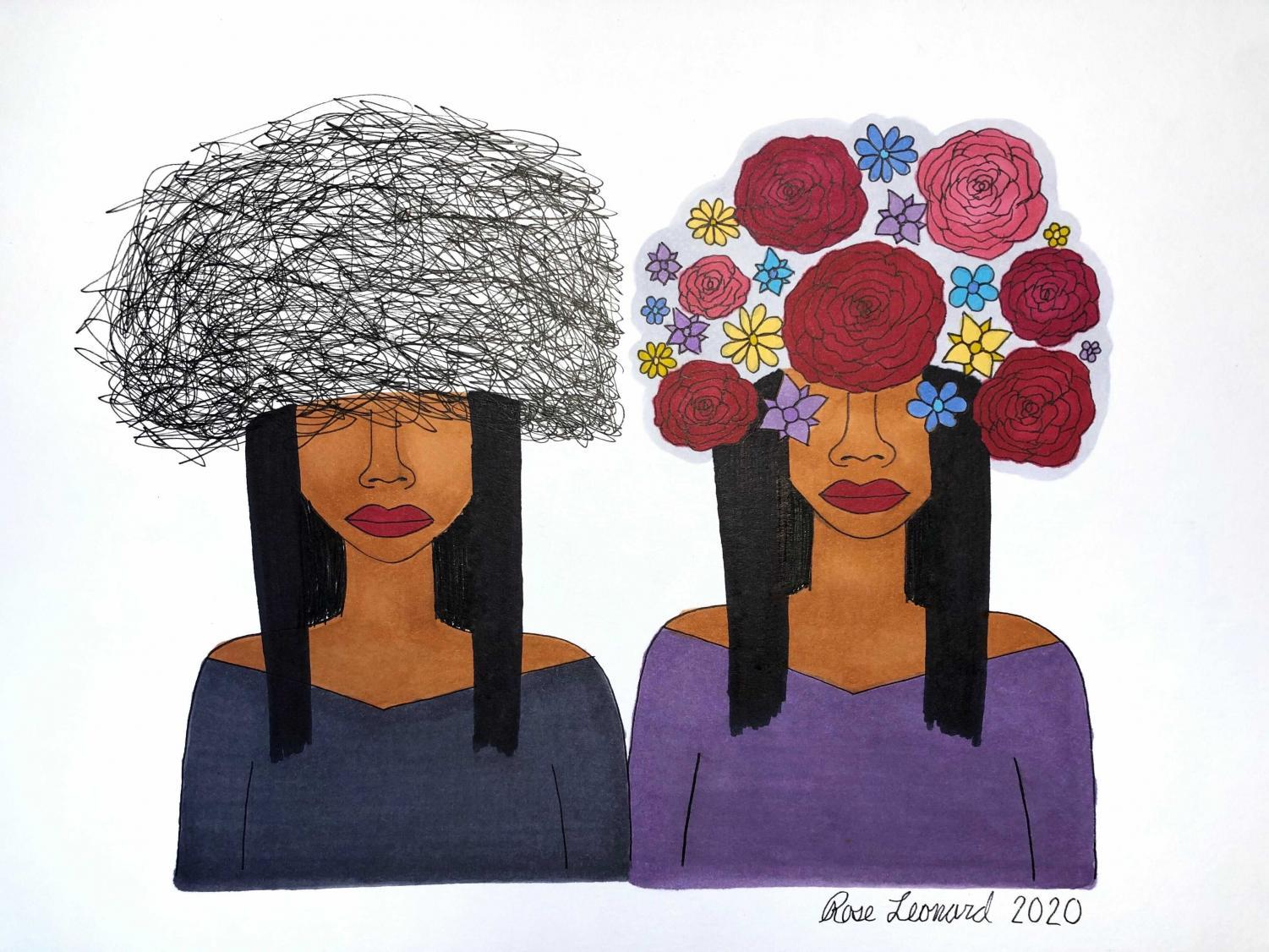This is a detailed artwork created by Rose Leonard in 2020, presented in a square format with a white and light bluish background. The image features two women, both with dark brown skin, standing side by side and portrayed in a cartoony style. Their long, straight black hair extends just past their shoulders, and they both wear the same shade of bold red lipstick.

The women wear identical off-the-shoulder tops with a wide V-neck. The woman on the left is dressed in a navy blue shirt, while the woman on the right wears a deep purple shirt. Each woman sports a distinctive hat that obscures the upper part of their face, hiding their eyes entirely.

The woman on the left has a jagged black and white hat that resembles a bird's nest, with swirls going everywhere. In contrast, the woman on the right wears a colorful floral hat adorned with red and pink roses, and small yellow, blue, and purple flowers. Some flowers even cover her eyes.

The artist's signature “Rose Leonard 2020” is inscribed in cursive black letters below the woman on the right, adding a personalized touch to the piece. The combination of vibrant colors, detailed patterns, and striking similarities between the women creates a visually captivating and harmonious composition.